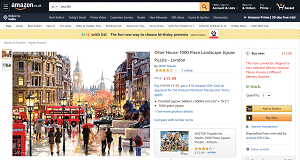The image displays a screenshot from an Amazon webpage. The top portion features a solid black banner with the Amazon logo in white, accompanied by a small orange underline. Adjacent to the logo are three small gray lines, indicative of a menu icon. A search box is prominently placed, with additional white text and a shopping cart icon to its right.

Below the black banner, there's a thin white line with legible text, followed by a beige-colored strip of text featuring black font. Within this beige strip, there is a small white box which contains a combination of blue text underlined in red.

The central focus of the image is a vibrant photograph of a bustling city street in England. Tall buildings surround the scene, and iconic red double-decker buses are visible. The street is populated with numerous pedestrians. Near the edge of the photograph, there is a red sign, as well as another sign displaying blue and black lettering.

On the right side of the image, a black headline draws attention. Below this headline are four gold stars, a price indicated in red, and a brief description in blue text. A small photograph is encased in a gray box close to this section. Further right, a tiny icon is accompanied by black text and a hint of pink. Below this, there are two small boxes featuring black text, followed by two brown boxes, and additional text in blue font.